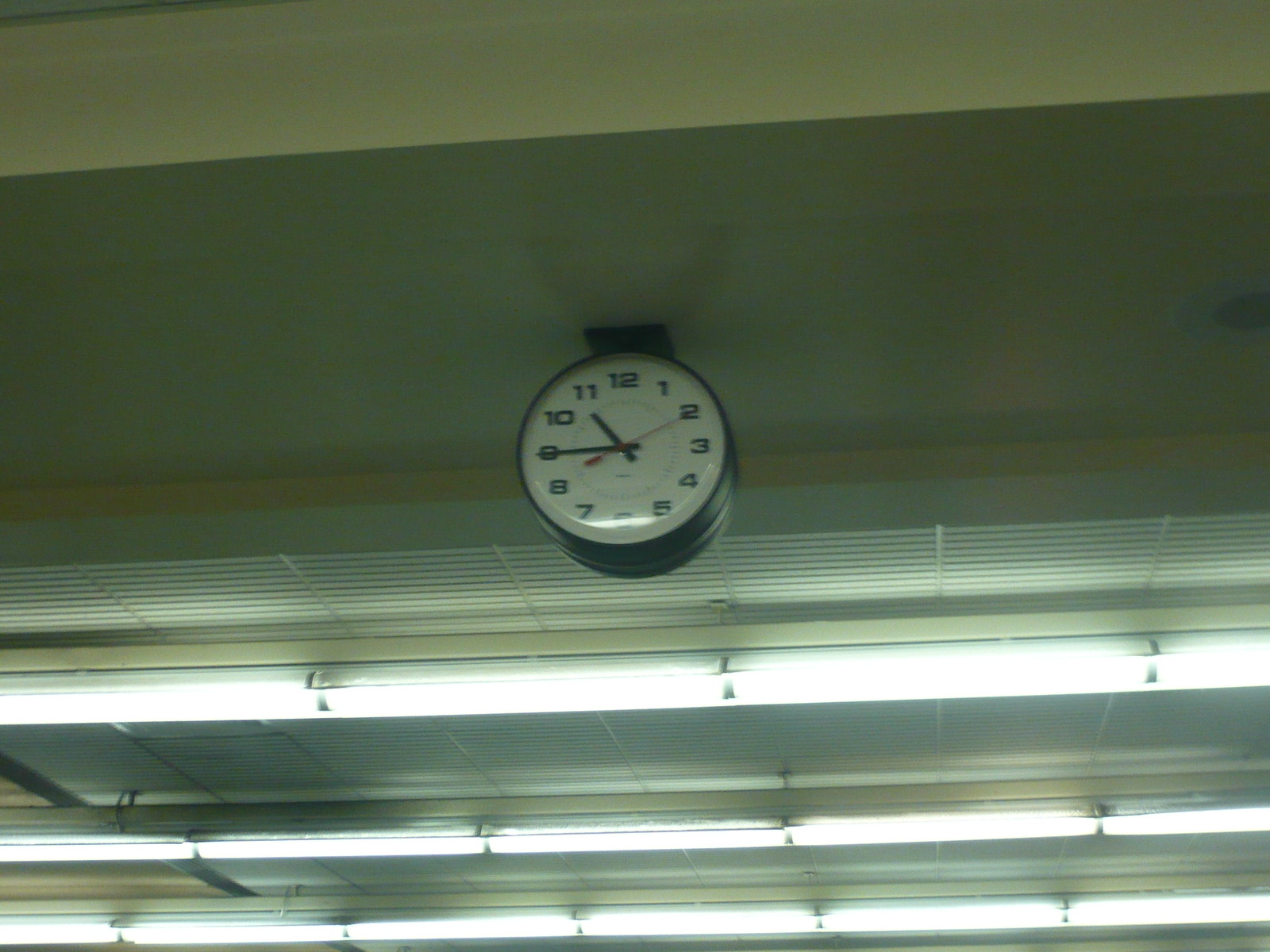The image captures a view from the floor looking up at a cement or concrete ceiling, likely in a cafeteria or similar large, utilitarian space such as a train station. Prominently featured in the foreground is a slightly out-of-focus ceiling clock with an angular black frame. The white clock face is marked by bold, black numbers and features black minute and hour hands. The hour hand points between 10 and 11, while the minute hand is on the 9, indicating a time of 10:45. Additionally, a thin, red second hand is visible, currently over the number 2. Surrounding the clock, the ceiling is adorned with three horizontal rows of generic-style fluorescent lights, each stretching from one side of the image to the other, attached to metal grids which suggest the presence of a drop ceiling. The ceiling itself exhibits alternating shades of dark gray and light gray, or possibly tan, adding a monotonous yet cohesive texture to the overall scene.